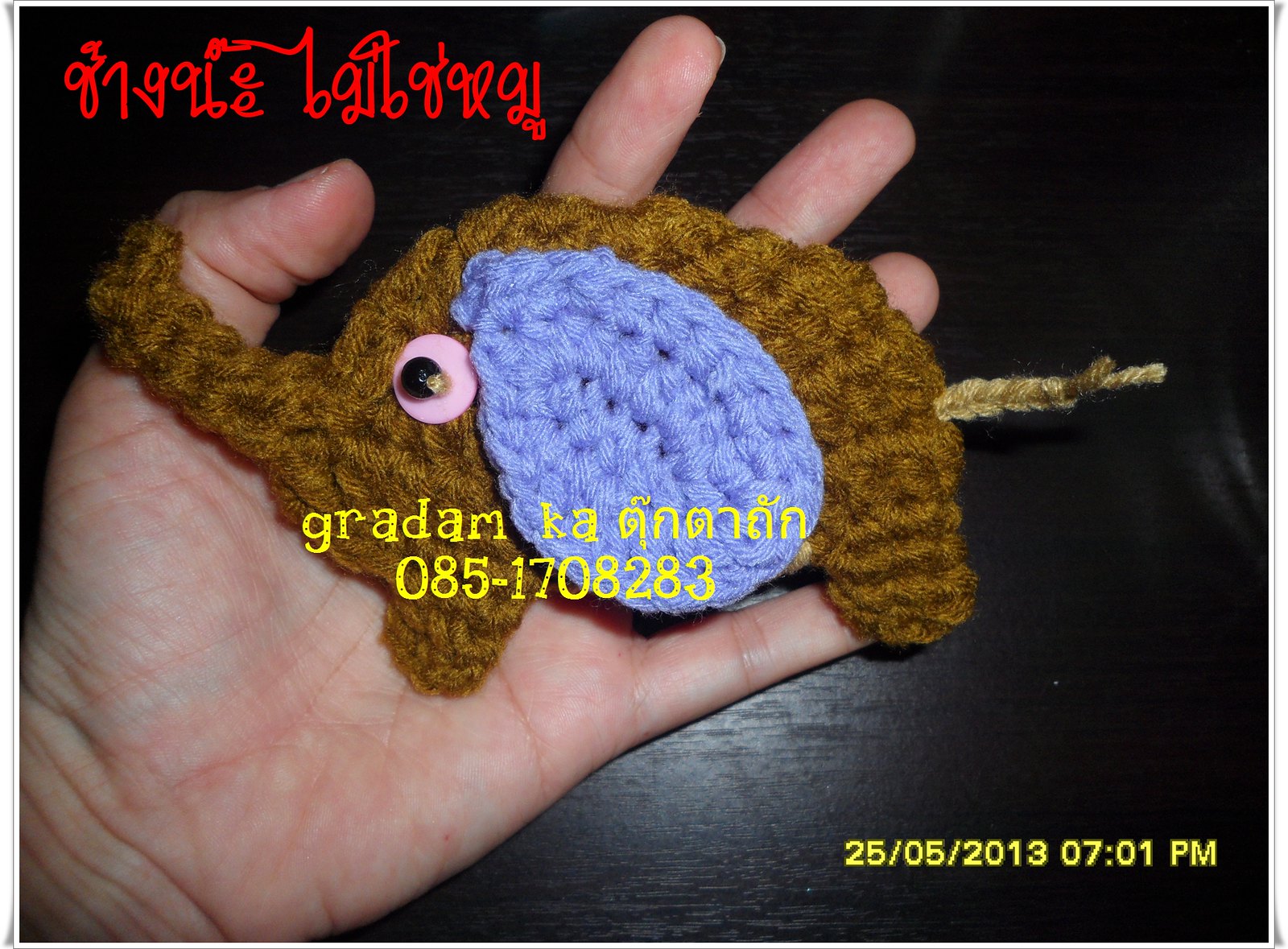A photo taken on May 25th, 2013 at 7:01 p.m. shows an outstretched left hand against a black background. The hand appears to be holding a hand-sewn or crocheted plushie resembling a small elephant. The elephant is primarily brown with a blue ear and a pink or possibly black bead serving as its eye. The plushie also features a light brown tail. In the top left corner of the image, there's some red text that is difficult to decipher, possibly in a foreign language, with parts reading "Kradom Ka" and other unreadable fragments.